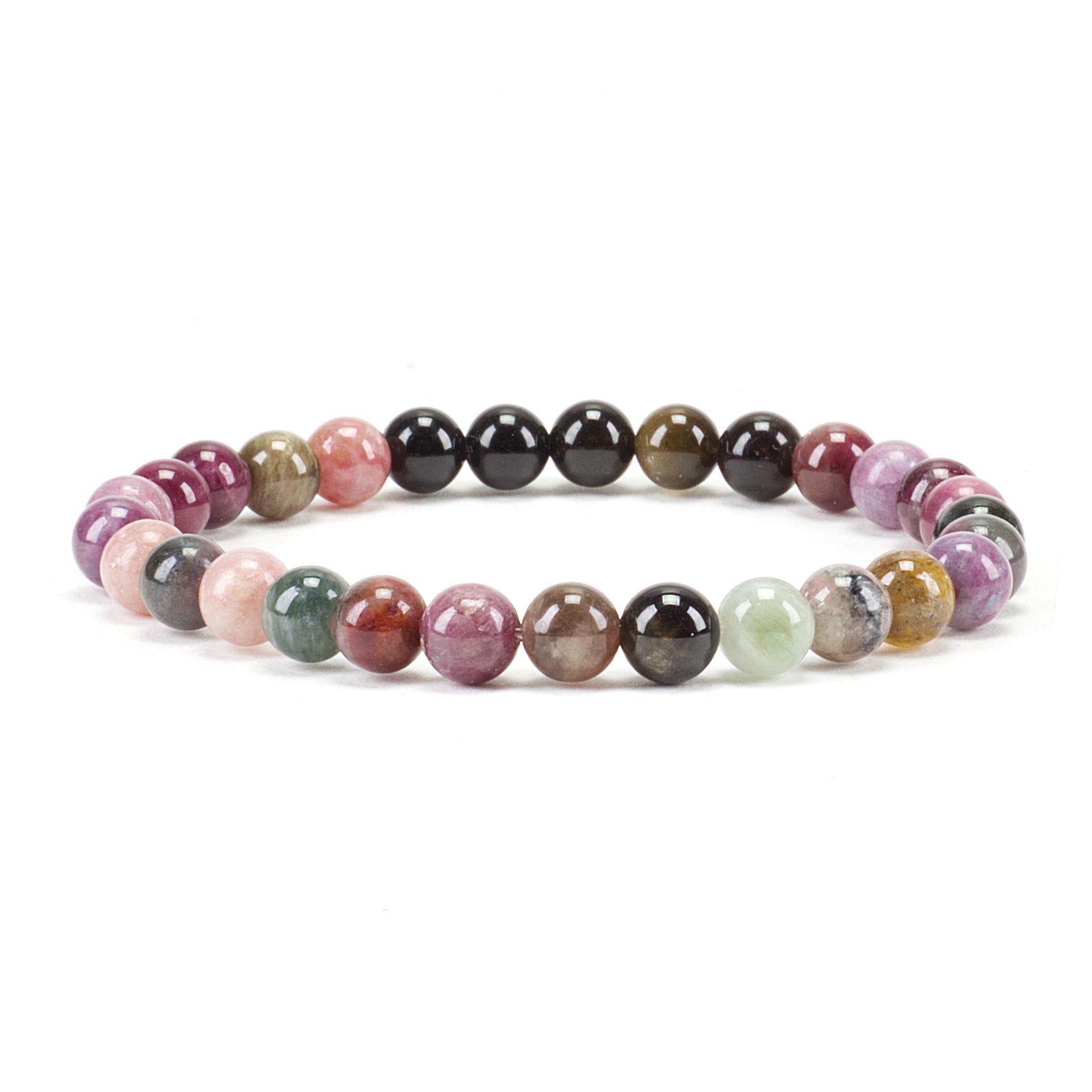This photograph showcases a single intricate bracelet composed of approximately 30 multicolored, glossy beads arranged in a circular shape, against a featureless white background. The beads, all uniform in size, span a diverse spectrum of colors including pink, various shades of purple, red, black, yellow, orange, green, and white, with several hues like root beer brown, sage green, forest green, peach, burgundy, and gray featuring distinct stone-like textures. Each highly polished bead reflects overhead light, creating white highlights on their tops and sides, and casting gray shadows beneath them, contributing to the professional and polished appearance suitable for an online product display.